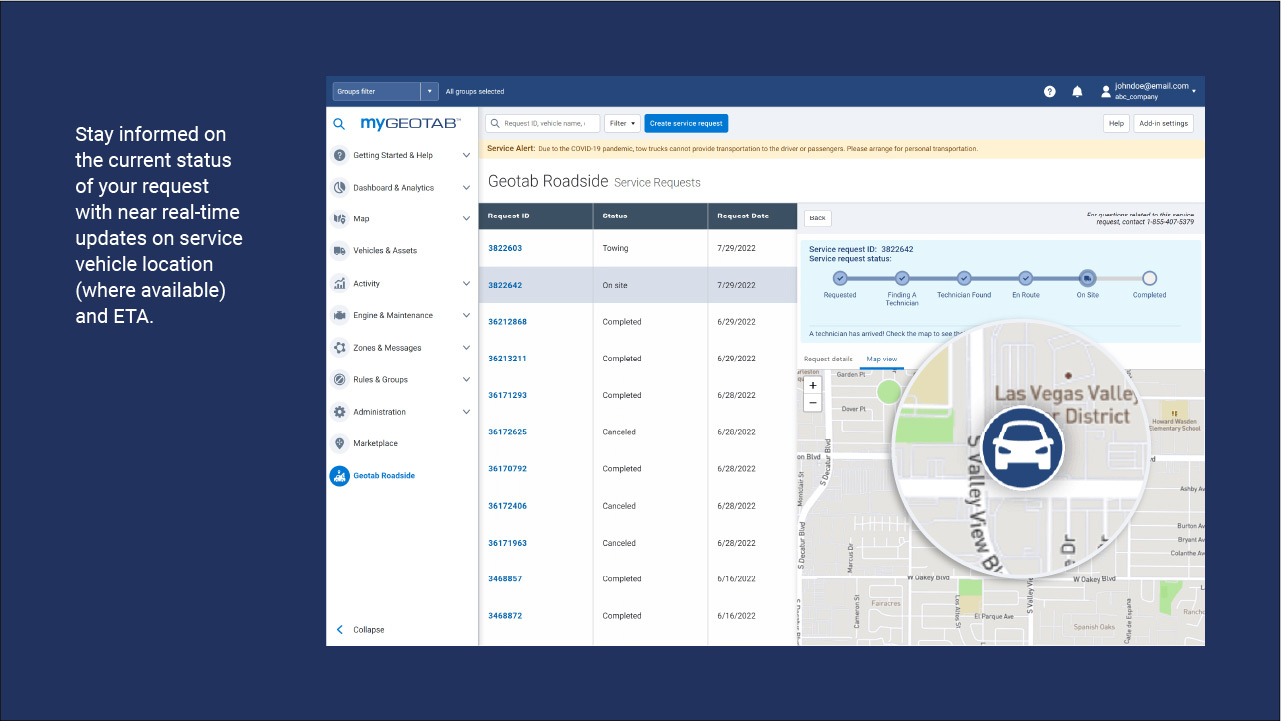The image displays a web page interface designed for tracking and managing vehicle service requests in near real-time. On the left side of the screen, a navigation panel includes various sections such as "Stay Informed," which offers updates on the current status of service requests, including the location and estimated time of arrival (ETA) of service vehicles where available. Additionally, there are options to filter groups, with "All Groups Selected" being highlighted.

The dashboard comprises several categories: "My Geotab," "Getting Started," "Help," "Dashboard and Analytics," "Map," "Vehicles and Assets," "Activity," "Engine and Maintenance," "Zones and Messages," "Roles and Groups," "Administration," and "Marketplace." A specific section titled "Geotab Roadside" is emphasized, providing service alerts pertinent to the COVID-19 pandemic. It mentions that, currently, trucks cannot offer transportation to drivers or passengers, advising users to arrange for personal transportation.

The main content area of the web page lists details of specific service requests. The first item, under "Geotab Roadside Service Request," has a Request ID of 3822603, and was initiated on July 29, 2022. The second entry, ID 3822642, is marked "On Site" with a request date of June 29, 2022. The third request, ID 36212868, shows a "Completed" status with a date of June 29, 2022.

All elements on the page provide comprehensive details enabling efficient tracking and management of vehicle service and maintenance requests.